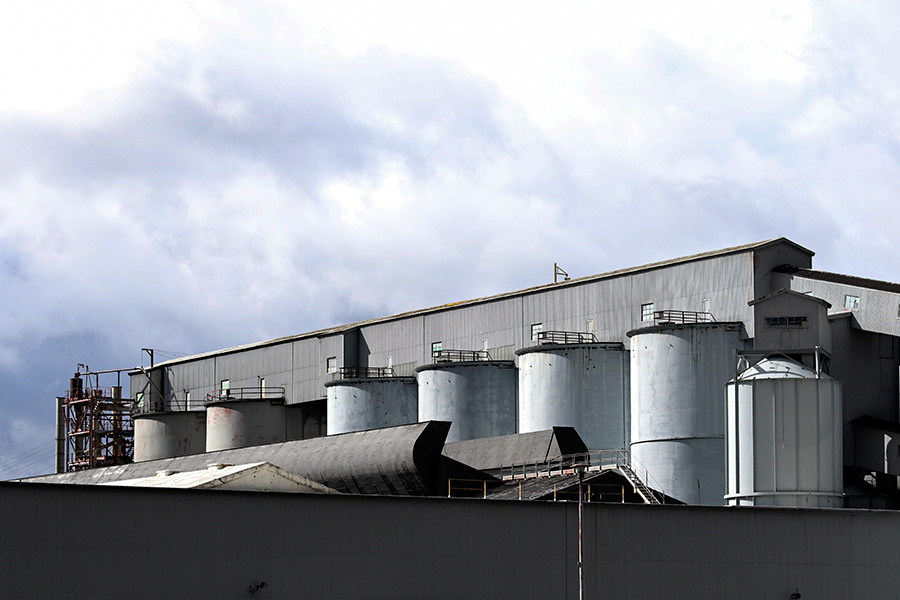The image depicts a close-up of an industrial complex that sprawls over a few stories. At the forefront, there are six large, round white cylindrical tanks or towers, which are likely used to store gas or water. These cylindrical structures have railings on top and are aligned in a row in front of a rectangular, multi-story gray building. The building is constructed with metal sides and features windows stretching across it, along with a gray metal roof. On the right side of the building, a large chute or ramp descends, appearing to be part of the industrial operations, potentially for transferring grains or another material. To the left, scaffolding is visible, adding to the industrial atmosphere. The entire setup seemingly sits atop another large building, also constructed from gray and steel materials, accentuating a cohesive industrial aesthetic. The background is dominated by a light blue sky filled with white clouds, adding a serene contrast to the heavy industrial elements below. In the foreground, there are two large, dark rolls that resemble tar or perhaps metal tunnels, adding further complexity to the scene.